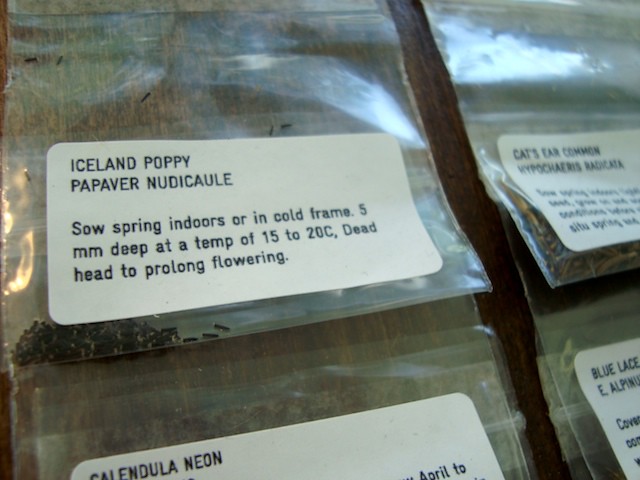This photograph showcases an assortment of seed bags, positioned against a wooden backdrop. The wooden surface adds a rustic charm to the scene, contrasting with the clear plastic bags that contain seeds. The seed packets feature prominently, filling most of the image without any specific centering. 

From left to right, the visible seed bags include:
1. **Iceland Poppy (Papaver nudicaule)** - This bag has a sticker providing detailed planting instructions: sow spring indoors or in a cold frame, 5mm deep at a temperature of 15 to 20 degrees Celsius; deadhead to prolong flowering.
2. **Calendula Neon** - Labeled "Calendula Neon," this bag is partially cut off but still recognizable.
3. **Cat's Ear Common (Hypochaeris radicata)** - This label reads "Cat's Ear Common" along with its scientific name.
4. **Blue Lace** - Positioned at the bottom right, this bag is labeled "Blue Lace E Alpha."

The bags are laid out flat against the wooden surface, with no single object centered, indicating a casual, perhaps store-like setting. The colors in the image are dominated by the natural brown of the wood and the clear and white elements of the plastic bags and labels, alongside some blank spaces.